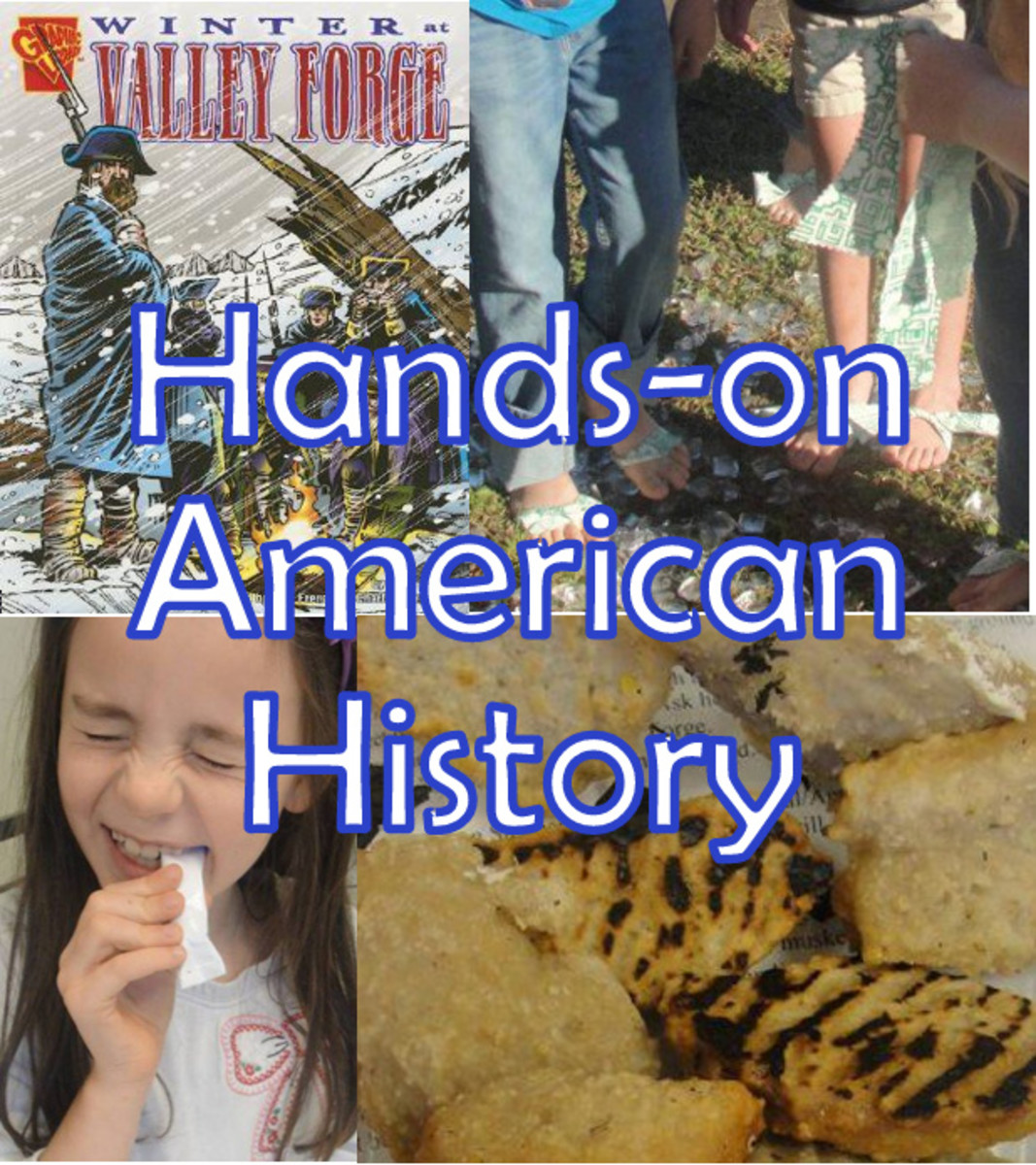This image consists of four illustrations and appears to be an advertisement or magazine cover titled "Hands On American History" in white text outlined in blue. The top left frame shows a cartoon-style illustration of four soldiers in blue cloaks and hats, huddled around a campfire in a snowy landscape, with streaks of falling snow. Above this, blue and red text reads, "Winter At Valley Forge." The top right frame shows the legs of three people standing on grass: one in blue jeans and white sandals, the next in beige shorts and white sandals, and the third in dark pants. The bottom left frame features a girl with long brown hair, a white shirt with a red design, holding a white object with her teeth and grimacing with her eyes shut. The bottom right frame is a close-up of grilled food that is beige and bready with black grill marks, possibly Johnny cakes or hardtack. Together, these visuals suggest an interactive and educational experience related to American history, possibly promoting a camp or event focusing on historical reenactments.